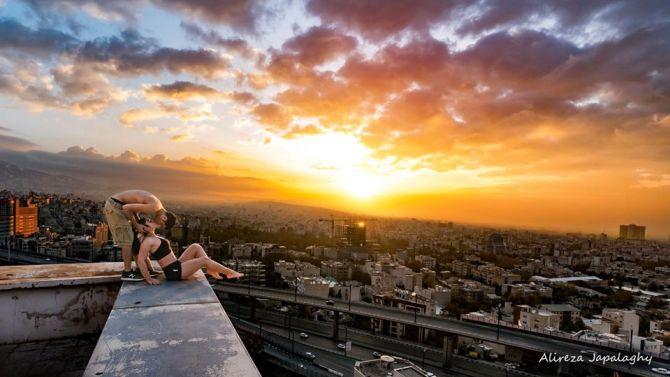In this stunning photograph by Alireza Chaplagya, a shirtless man wearing khaki shorts and black tennis shoes leans over to kiss a young woman. She sits on the edge of a tall, rusty, distressed rooftop, her feet dangling over, clad in black shorts and a black bra top. The couple is perched on the left side of the image, sharing a tender moment against a breathtaking urban backdrop. Beyond them, a sprawling city skyline stretches out, with towering skyscrapers, assorted apartment buildings, and a bustling highway teeming with cars. The sky steals the show with its mesmerizing hues—clouds bathed in the rich orange glow of the setting sun merge seamlessly into blue sky on the left. The copyright in white print, "Alireza Chaplagya," is elegantly placed in the bottom right corner, adding a final artistic touch to this captivating scene.